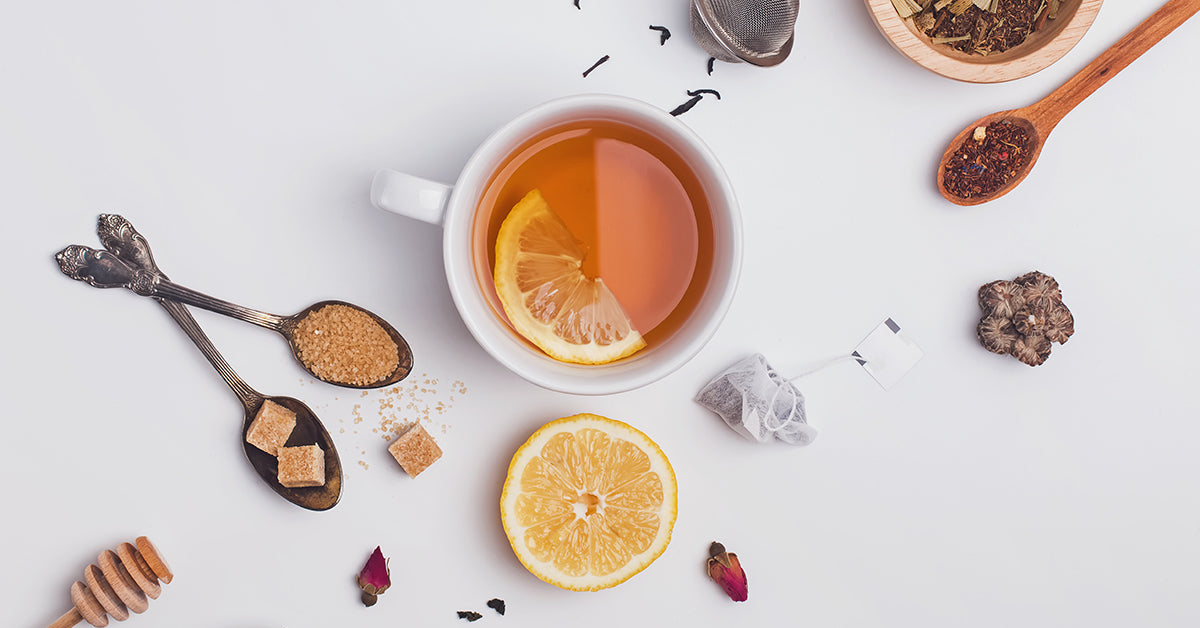This overhead photo, taken on a white surface, showcases a visually rich tea-themed arrangement. At the center is a cup of tea with an orangish-brown hue, partly immersed in it is a half slice of lemon or orange. Surrounding the cup are various tea accompaniments meticulously positioned. 

To the right of the cup sits a small wooden bowl filled with loose tea leaves, accompanied by a mesh tea strainer and a wooden spoon, also laden with dried tea leaves. Adjacent to the bowl are dried pink flowers, and a spoon with seasonings. Farther to the right, a tea bag and a purple flower add to the assortment of ingredients.

On the left side of the cup is another half slice of a citrus fruit and two spoons placed side by side; one holds brown turbinado sugar, while the other contains two sugar cubes, with additional sugar crystals scattered below. A single sugar cube lies on the surface, surrounded by loose bits of brown sugar. 

In the bottom left corner of the image, a spiraled honey dipper awaits use, emphasizing the tea’s sweetening options. The combination of these elements against the pristine white backdrop makes for a harmonious and inviting composition.